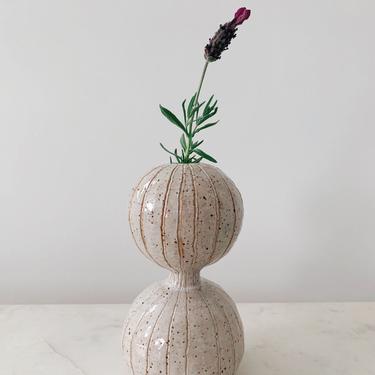In the image, a unique vase resembling the shape of two pumpkins stacked atop one another with a narrow gap between them, sits on a light marble table speckled with gray and black. The vase, primarily white with intricate pink lines and occasional black and gray flecks, serves as an elegant centerpiece. From the vase, a singular stalk of green leaves emerges, ascending halfway up before giving rise to a dark blackish-purple flower bud. The flower, not yet fully bloomed, features maroon and pink streaks running down its center towards the tip. The backdrop consists of a plain gray wall, enhancing the muted and sophisticated aesthetic of the scene, with no other elements present in the photograph.